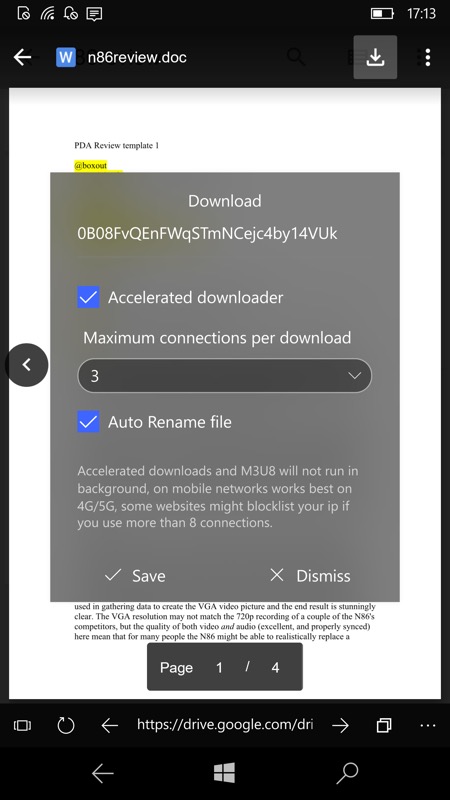The image features a black rectangle with various symbols and icons. In the upper left corner, several icons can be seen, including what appears to be a Wi-Fi signal, a bell with a line through its circle, and a speech bubble with lines inside. On the upper right corner, there's a partially filled battery icon with the number "713" next to it.

Below these icons, there's a white arrow pointing to the right. Adjacent to it, there's a blue square with a white "W" inside, followed by white text. Beside the text, there’s a gray square with an arrow pointing down into what resembles a box, followed by three white dots in a line.

A white rectangle below these elements contains various text, including a portion highlighted in yellow. Inside this white rectangle, there's a gray rectangle labeled "Download" accompanied by several letters and numbers.

Further down, a blue square with a white check mark labeled "Accelerated Download" or "Maximum Connections per Download" is displayed. Another gray rectangle, with bulges on both sides, is marked with the number "3" and an arrow pointing down.

Another blue square contains a white check mark and is labeled "Auto Rename File," with some text below it. Beside these, a check mark labeled "Save" is followed by an "X" labeled "Dismiss."

Below these options, in black text, a dark gray rectangle is labeled "Page 1-4." Adjacent to this are several symbols: a square with lines on its sides, almost complete circle with an arrow inside, a left-pointing arrow, a website label, a right-pointing arrow, two overlapping squares, and three dots.

Towards the bottom left, there's another right-pointing arrow, a Windows symbol, and a magnifying glass icon.